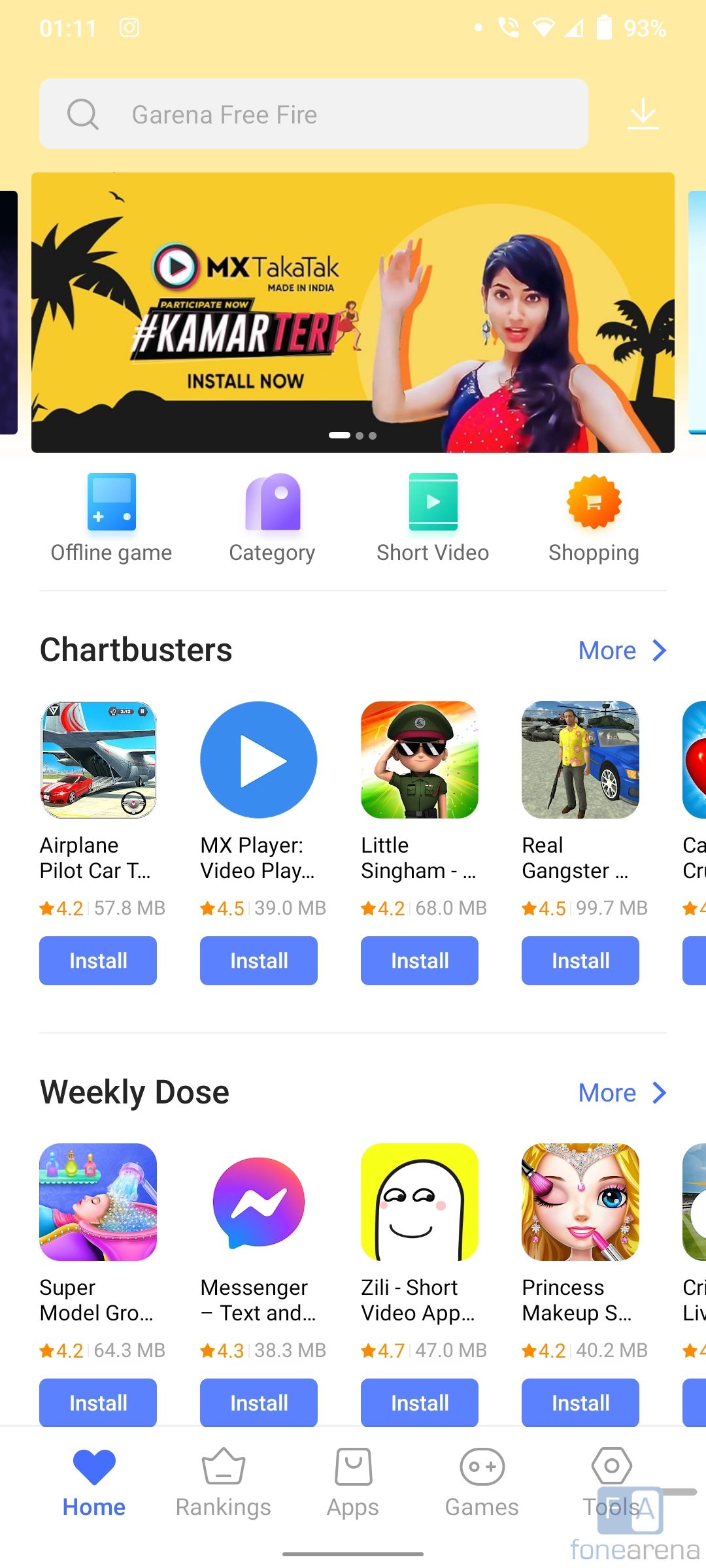This image appears to be a screenshot of a cellphone displaying an app store interface. The layout predominantly features a white background with various app categories and options to either install or purchase apps. Each app listing includes a thumbnail image, a blue "Install" button, user ratings denoted by stars (e.g., 4.2, 4.5), and the app size in megabytes (e.g., 54 MB, 57.8 MB).

At the top of the image, there is an advertisement featuring an Indian woman in a red dress with her hand raised. This ad encourages users to install an app called "Hashtag Kamar Tech" with a prompt "Install now."

Below this advertisement, multiple categories are displayed, including "Offline Games," "Short Videos," "Shopping," "Chart Busters," and "Weekly Dose." 

The "Chart Busters" category includes apps like "Airplane Pilot Car Game," "MX Video Player," "Little Singham," and "Real Gangster." 

The "Weekly Dose" category features apps such as "Supermodel Grow," "Messenger Text and App," "Zilli Short Video," and "Princess Makeup."

At the bottom of the screen, navigation buttons are visible, including "Home," "Rankings," "Apps," "Games," and "Tools." The interface is currently on the "Home" page.